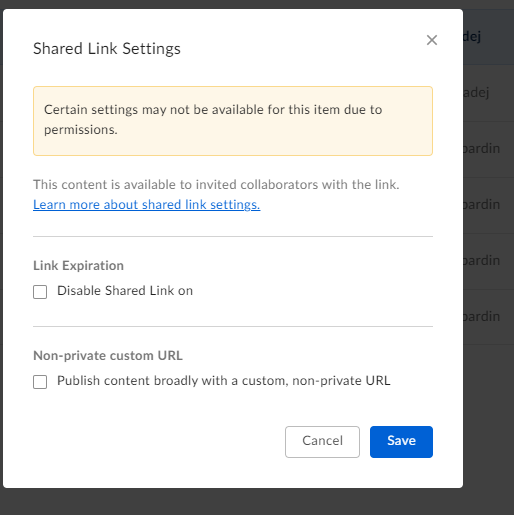The image features a white, vertical rectangular overlay positioned atop a darkened background image. The background shows partially obscured text running along its right edge, partially cut off by the white overlay on top. The darker background image has a subtle shade over it, giving it a muted appearance.

At the top of the white overlay, the large black text reads, "Shared Link Settings," accompanied by a gray 'X' icon on the far right side. Below this heading, a yellow rectangular horizontal strip, outlined in golden color, contains the black text, "Certain settings may not be available for this item due to permissions."

Underneath the yellow warning strip, the black or possibly gray text states, "This content is available to invited collaborators with the link." Directly below this, a bright blue link, underlined, reads, "Learn more about shared link settings."

A light gray horizontal line separates the initial section from the next. The following section begins with gray text reading, "Link Expiration," next to an empty checkbox labeled "Disable Share Link."

Another thin gray line divides this section from the subsequent one, which includes the gray text, "Non-Private Custom URL." This is followed by an empty checkbox and the instruction, "Publish content broadly with a custom non-private URL," also in gray text.

At the bottom of the overlay, there's a "Cancel" button with a white background, light gray border, and black text. Adjacent to it is a horizontally-aligned "Save" button, colored blue with white text.